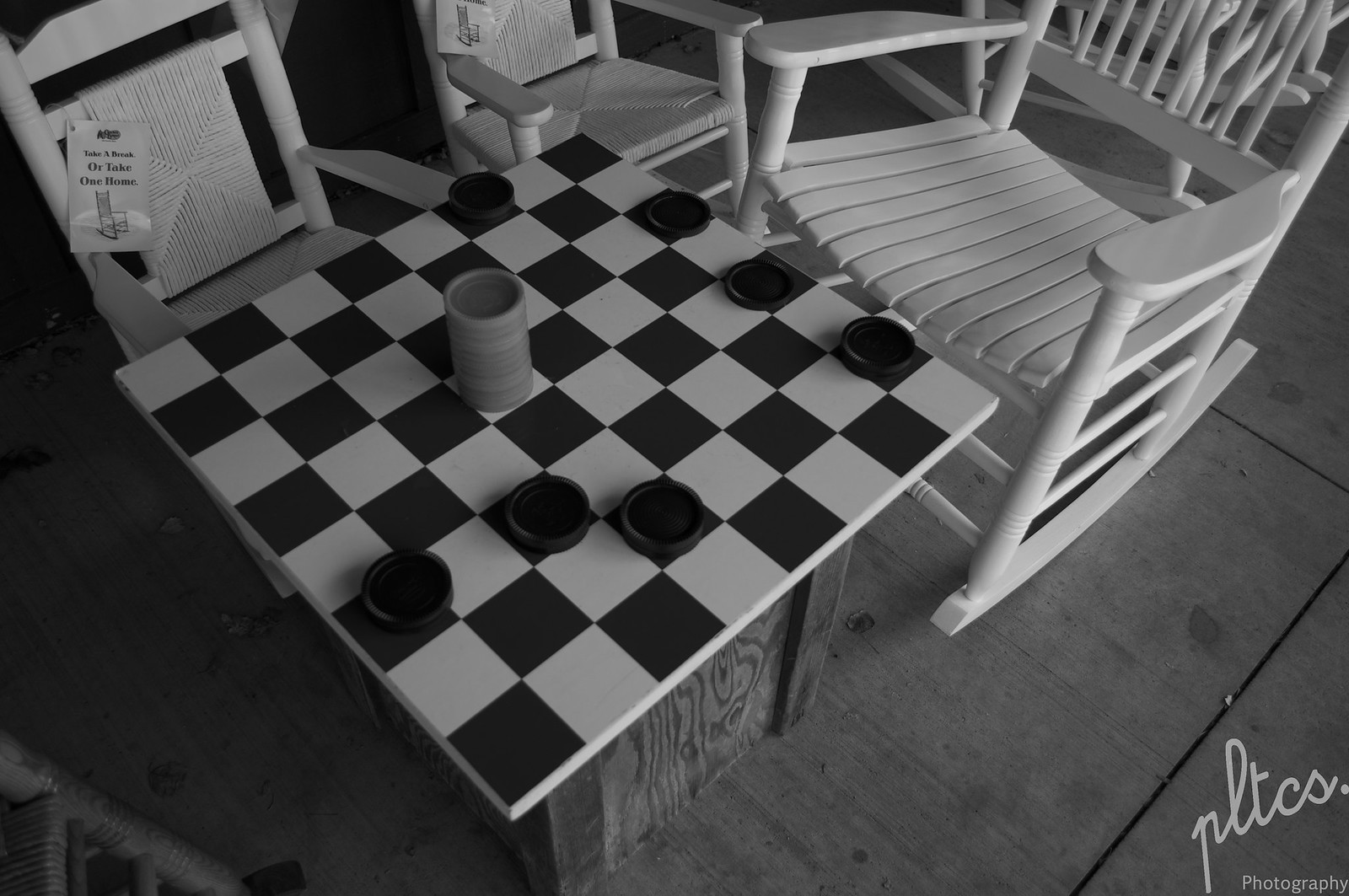In this black and white photograph taken from a slight overhead angle, we see a checkers board oriented as a diamond, with its corners pointing to the top, bottom, left, and right. The board features both black and gray checkers, with several pieces clustered towards the upper right and center of the board. Notably, some gray checkers are stacked on one of the white squares in the middle. The board itself is set atop a rustic wooden shipping crate. 

To the upper parts of the board, there are several chairs positioned on wide wooden flooring. A white wooden rocking chair is prominently featured to the right, reflecting a glossy finish. Additionally, to the upper left, there is a small wicker chair with a tag that reads "take one home," indicating the scene might be in a Cracker Barrel restaurant sales area where customers can relax and play checkers. The photograph's lower right corner includes a signature followed by the word "photography," suggesting it might be part of an exhibit. Overall, the image captures the quaint and inviting atmosphere of a Cracker Barrel restaurant, complete with cozy white rocking chairs and a classic checkers game.